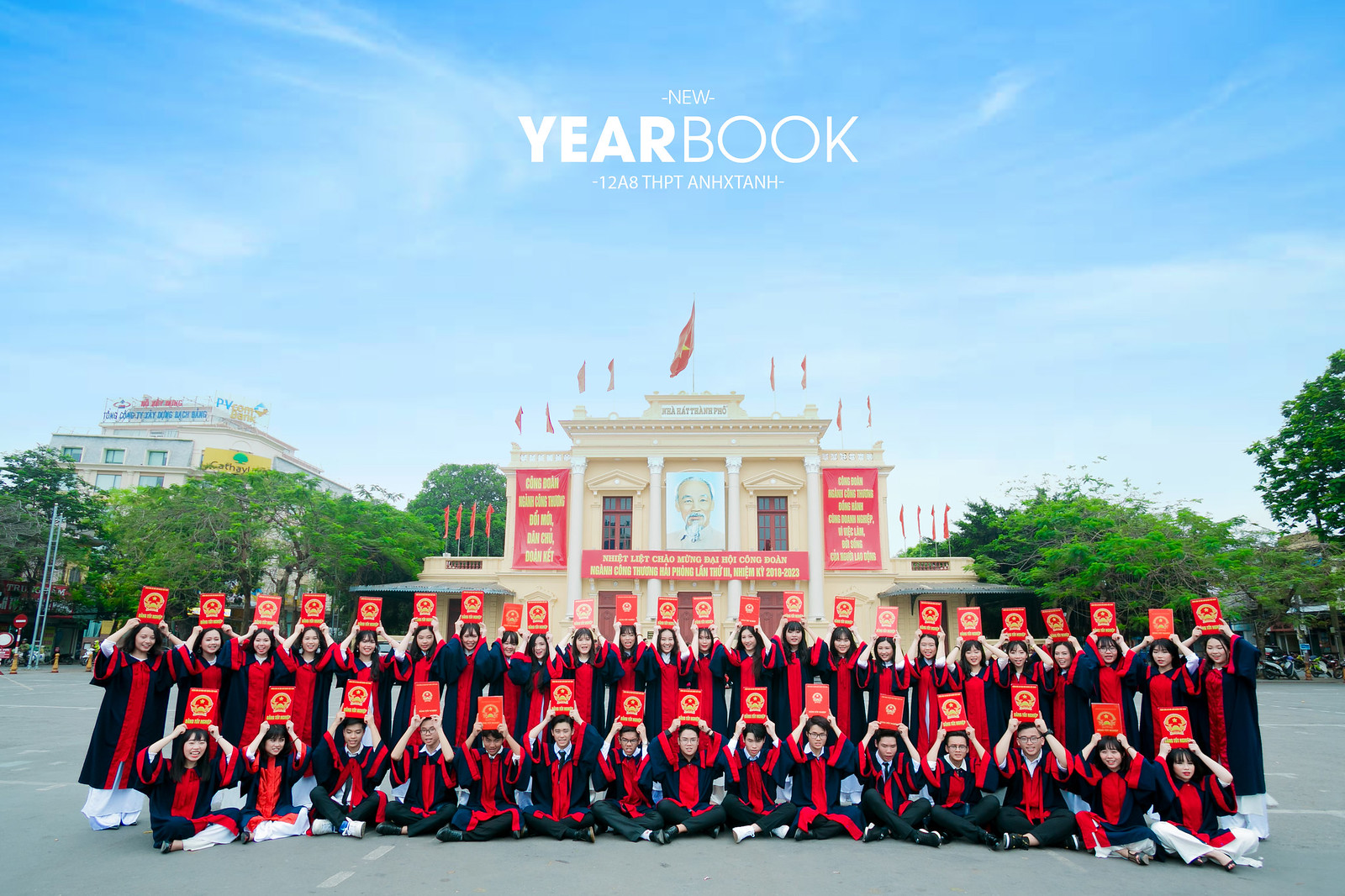This vibrant image captures a group of nearly 50 newly graduated students of Asian descent. They are dressed in red and black graduation robes and hold red diplomas with gold writing above their heads in a proud display of their achievement. The students are arranged in two rows, with the first row sitting on the ground and the second row standing behind them. Interestingly, the top row consists predominantly of women, while the bottom row has a mix of both men and women. The background showcases a white, ornate school building adorned with red banners on either side and a horizontal red sign in the middle. The scene is set under a clear blue sky with minimal clouds, and framed by lush greenery and tall trees flanking the building. Above the building, in bold letters, it reads "New Yearbook 12A8THPTANXTANH."